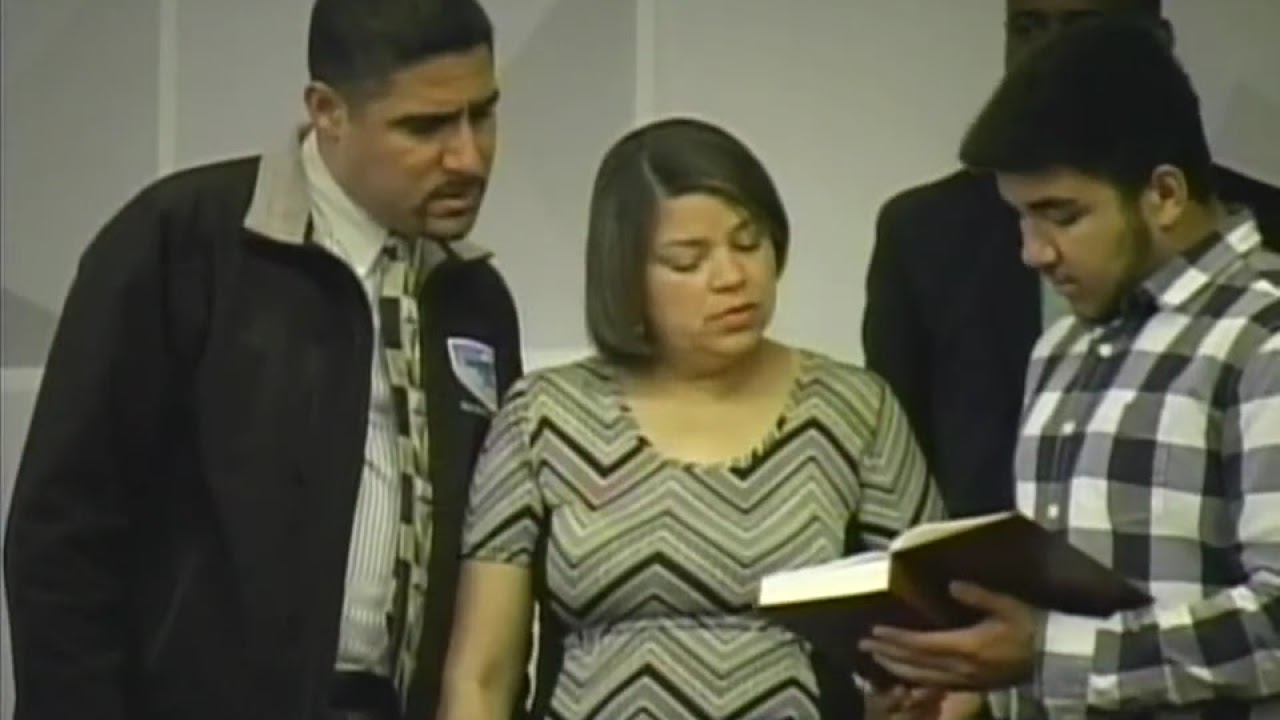The image depicts a group of four people intently reading a book, which appears to be a Bible, suggesting they are in a church setting. The main focus is on a man with short brown hair and a slight beard, wearing a black, white, and gray plaid shirt. He is holding the book open to a specific page. To his left stands a woman with short brown hair, dressed in a black, white, and gray striped dress. She is closely examining the book along with the man. To the woman’s left is another man, distinguished by his dark jacket, white shirt, and a black and brown tie; he has a goatee and brown hair. Positioned slightly behind the woman, this man is also looking down at the book. A fourth person, a man partially visible in the background, seems to hover around the group, further hinting at the communal nature of this gathering. The backdrop features a flat grayish design, aligning with the solemn and formal atmosphere suggested by the attire of the individuals. All four individuals are deeply engaged with the contents of the book, which they crowd around, taking up most of the frame.